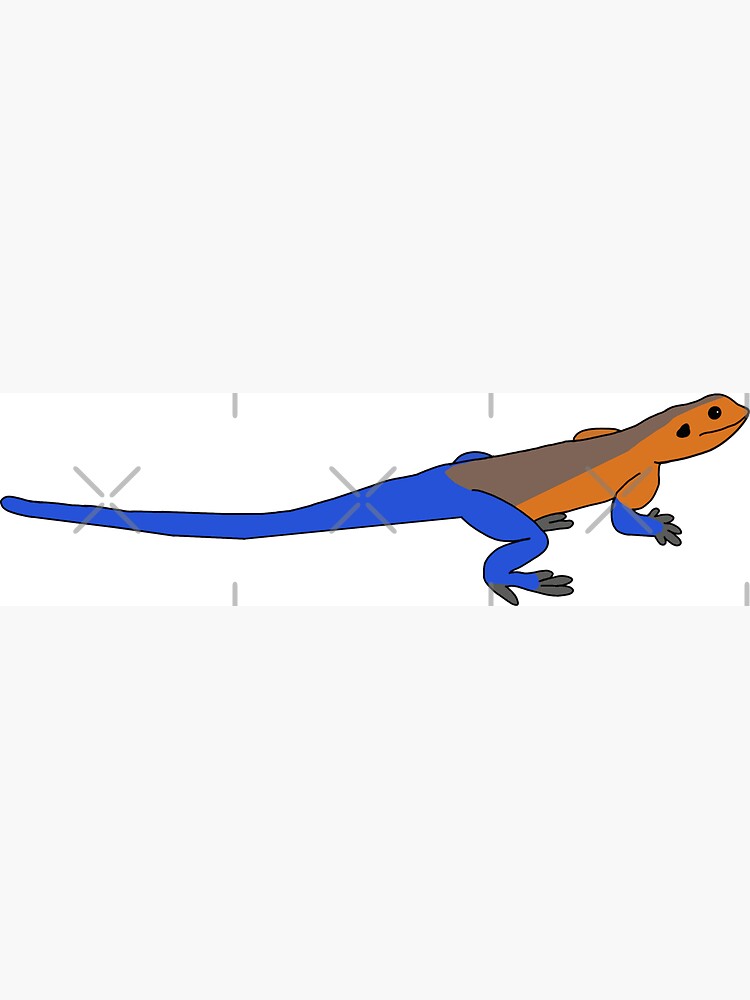In this digital artwork, the centerpiece is a detailed drawing of a lizard, depicted from a side profile. The lizard has a striking long blue tail that stretches westward, alongside its blue legs that appear longer and more curved towards the back than the front. The lizard's body is painted in a light amber-brown gold color, with a solid brown hue adorning the top of its head extending towards its tail. The lizard’s closed mouth is depicted as a straight line, and its eye is rendered black. Additionally, there's a visible opening on the side of its head, representing its ear. The image also features small gray X's, acting as watermarks, with three placed across the lizard’s body and one over its foot.